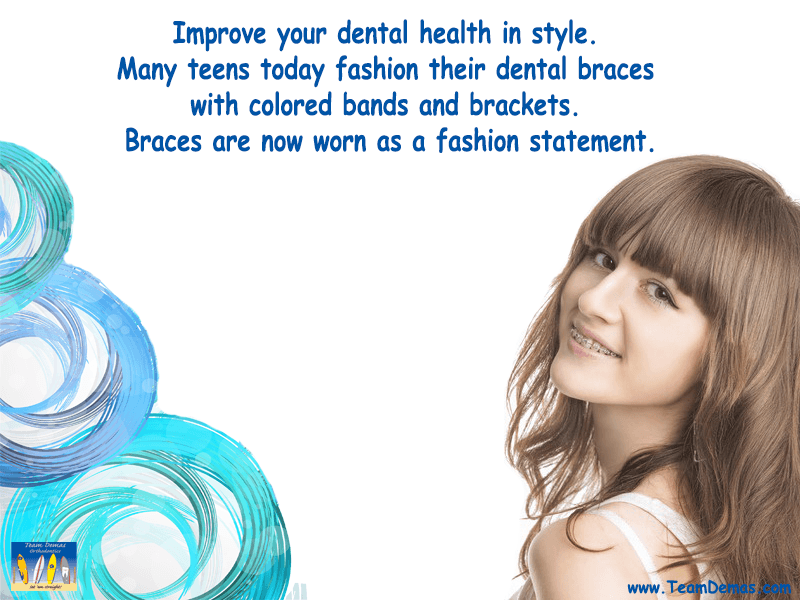The image features an advertisement for dental braces. At the top, in vibrant blue text, it says, "Improve Your Dental Health in Style." It emphasizes how many teens today use colored bands and brackets to make their braces a fashion statement. On the right side of the image, there is a real photograph of a young girl with long, light brown hair and bangs. She is smiling, revealing her braces, which appear transparent. The girl is wearing a white tank top and has her head slightly turned as if posing for the camera. On the left side of the ad, there are artistic swirls in varying shades of blue, from turquoise to deep blue, creating a dynamic visual element. At the bottom of the poster, the website "www.teamDMAS.com" is displayed in blue text. In the bottom left corner, there's also a small symbol featuring yellow and brown-gray surfboards, adding a playful touch to the design.